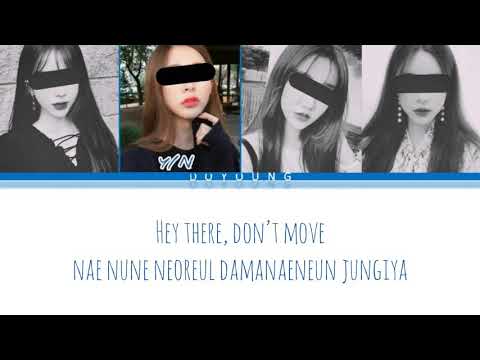The image appears to be an advertisement featuring a sequence of four images of women. At the top, there is a thin, horizontal black rectangle. Below this, the four pictures are aligned in a row. All four images depict women with long dark hair, except for the second one from the left, which is in color and features a woman with long light brown hair and pale skin. Each woman has a black slash covering her eyes. The bottom of the image features a white text box with blue letters that reads, "Hey there, don't move," followed by additional text in a foreign language. Surrounding the pictures is a blue rectangle, and at the bottom, there is another black horizontal rectangle completing the border. The overall effect is a striking, stylized arrangement that captures attention.